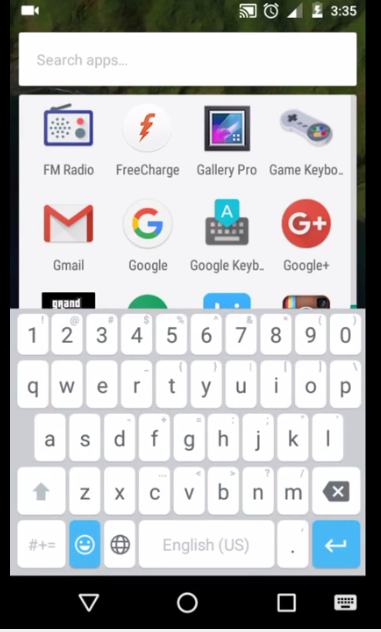This screenshot captures the interface of an Android smartphone in portrait orientation. At the top of the screen, details like the clock, a battery icon showing charging status, and various notification symbols are visible. The screenshot showcases the app drawer, which displays all the installed apps, visible after swiping up from the bottom of the screen. Dominating the lower half of the screen is the on-screen keyboard.

Notably, the navigation bar at the bottom features three distinct digital buttons: a triangle pointing downwards on the left, a circle in the center, and a square on the right, all of which are characteristic of Android devices. Apple's iOS generally does not utilize this three-button system.

The screen displays several Google-related apps, reinforcing the likelihood of it being an Android device. These include Gmail, Google, Google Keyboard, and Google+. Additional clues suggesting this is an Android phone come from the presence of a game keyboard icon, which indicates sideloaded gaming apps—a common practice among Android users but less so among iOS users. Overall, the combination of the navigation buttons, the visible apps, and the keyboard strongly indicates that this is an Android phone.